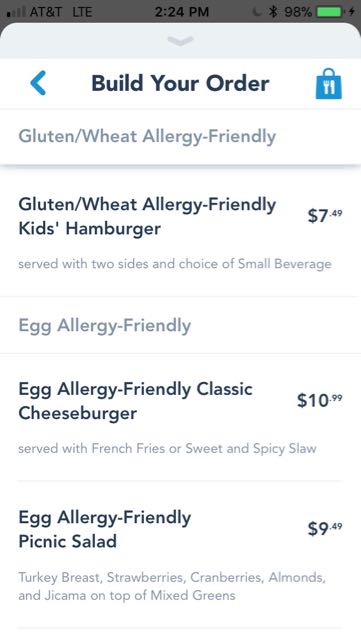This screenshot, captured on an older iPhone at 2:24 p.m., displays a page from a food ordering app that allows users to customize their delivery orders with specific dietary preferences. At the top, the page prompts users to "Build Your Order," followed by an icon of a blue shopping bag adorned with a fork and knife. The app highlights its ability to accommodate various allergies, ensuring food safety for those with dietary restrictions—a feature not commonly offered by many apps.

The curated options include:

- **Gluten/Wheat Allergy Friendly Kids Hamburger**: Priced at $7.49, this meal is designed for children with gluten or wheat allergies. It is served with two sides and includes a choice of a small beverage.
  
- **Egg Allergy Friendly Classic Cheeseburger**: This $10.99 option is tailored for individuals with egg allergies. The cheeseburger is served with a choice of French fries or a sweet and spicy slaw.

- **Egg Allergy Friendly Picnic Salad**: For $9.49, this salad caters to those with egg allergies and features turkey breast, strawberries, cranberries, almonds, and jicama atop mixed greens.

The app's focus on allergen-friendly options demonstrates its commitment to providing inclusive food choices for all customers.